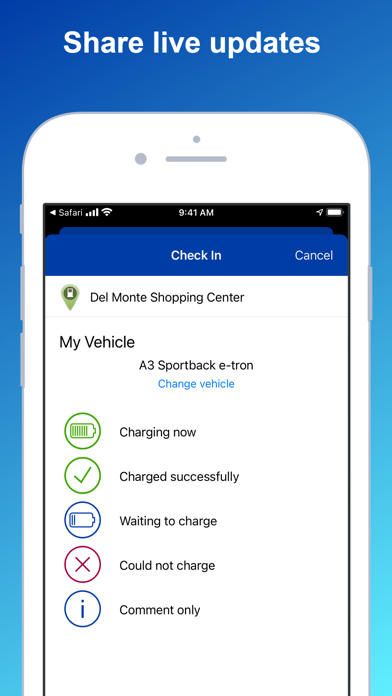The image depicts a smartphone screen against a gradient background that transitions from blue at the top to teal aqua at the bottom. The phone displays full signal strength and shows the time as 9:41 a.m. The top bar of the screen, featuring a black background, reads "check." Below this, a notification banner with a blue background displays "Check In."

The primary interface on the screen, set against a white background, shows detailed information about the Del Monte Shopping Center. Listed beneath this is "My Vehicle," identified as an "A3 Sportback e-tron." There's an option to "Change vehicles" in small blue text.

A status section details the vehicle's charging progress:
- A battery icon within a green circle indicates "Charging Now," accompanied by a checkmark and the text "Successfully charged."
- A blue circle with a blue battery icon indicates a status of "Waiting to charge."
- An icon of a round circle with an X through it states "Could not charge."
- Another blue circle with an 'i' symbol denotes "Comment Only."

This comprehensive display implies the screen is monitoring the status of an electric vehicle's charging process in the shopping center's parking lot.